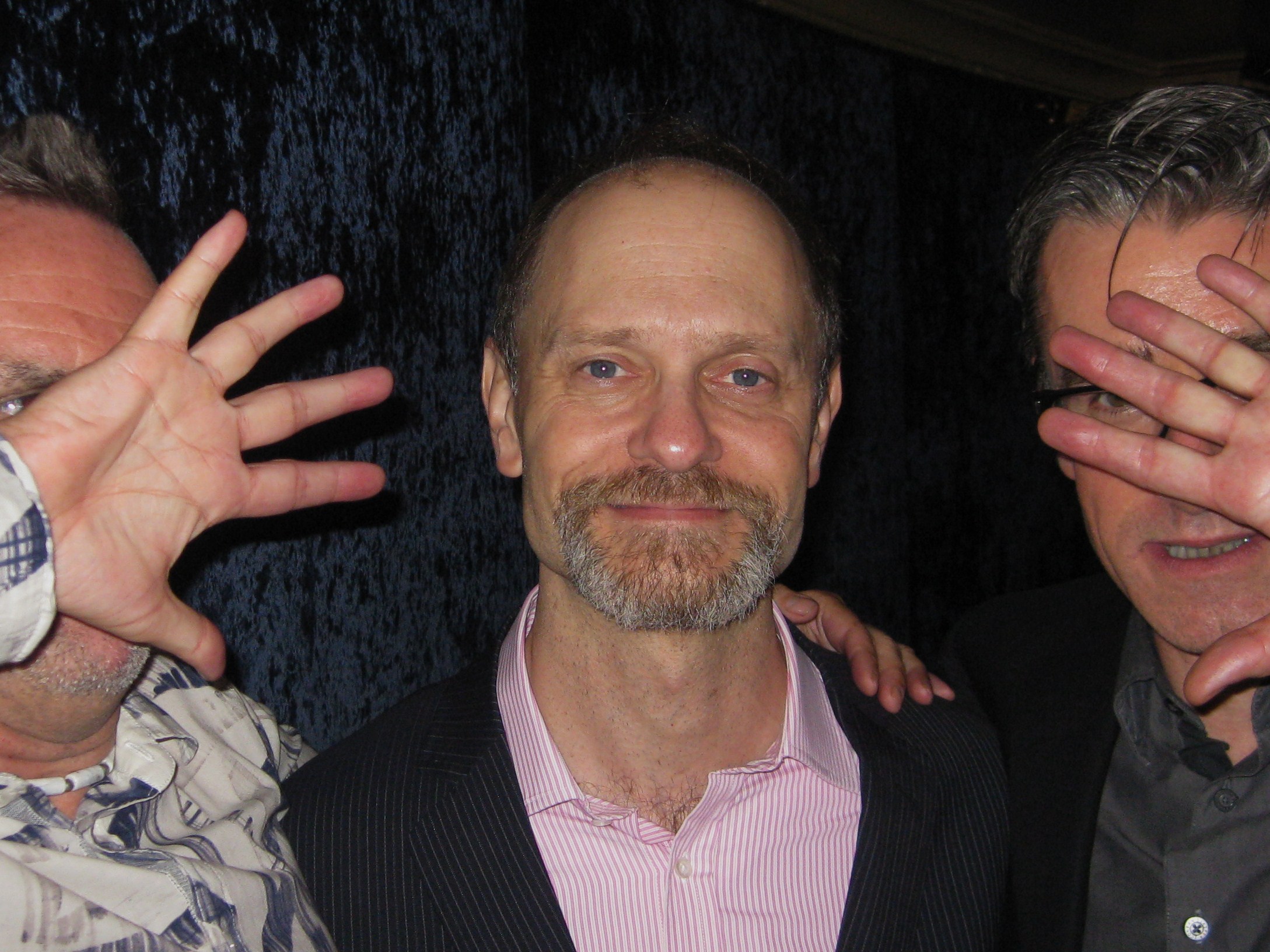The photograph captures three men from their upper chest upwards, positioned against a backdrop of luxurious blue velvet fabric. The central figure, a balding man with sparse brown hair, sports a graying mustache and beard, and is dressed in a black and gray striped business coat over a red and white striped shirt with the top button undone. He gazes forward with a subtle, closed-mouth smile. On either side of him, the other two men have their faces obscured by their hands. The man on his right wears a gray button-up shirt with the top button undone, beneath a black business coat and black-rimmed glasses. The man on the left dons a long-sleeve button-up shirt with blue plaid designs and a red and white beaded necklace. Their presence and attire, coupled with the rich blue background, create a striking and engaging composition.